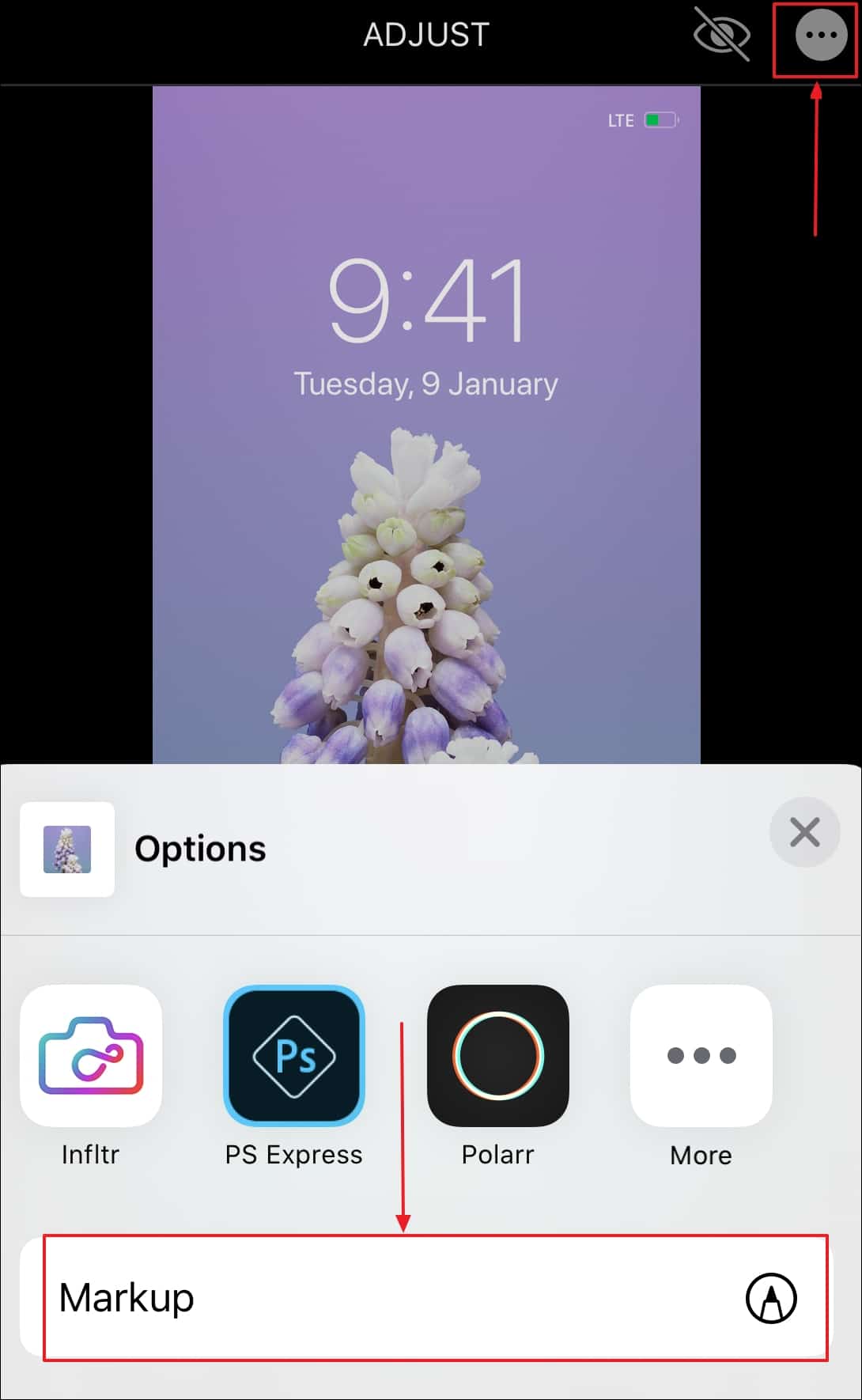The image appears to be a screenshot from a mobile phone displaying a partially edited photograph of beautiful, partially bloomed flowers. Dominating the image is a cluster of delicate flowers, each with purple and white petals—transitioning from a rich blend at the base to pure white at the tips. The flowers, set against a serene lavender background, seem to be closed, suggesting they aren't fully bloomed yet. 

Front and center, the time is prominently displayed as 9:41, and the date is noted as Tuesday, January 9. The screen is further adorned with typical smartphone elements: an LTE signal indicator, a battery icon, the word “ADJUST” positioned at the very top center, and a crossed-out eye symbol to the right.

Amid the editing interface of a photo application, there's a conspicuous white circle featuring three dots, encased in a red outline with an upward-pointing arrow, presumably a control button for further adjustments. Below this, several options are presented: “PS Express,” “Polarr,” and “MORE,” each in their own white square. There's also an “X” button situated on the right-hand side, perhaps to close the editing menu.

In the background of a light gray interface, additional editing tools are available. A red markup box features the word "MARKUP” alongside a pen or pencil icon, indicating further customization options.